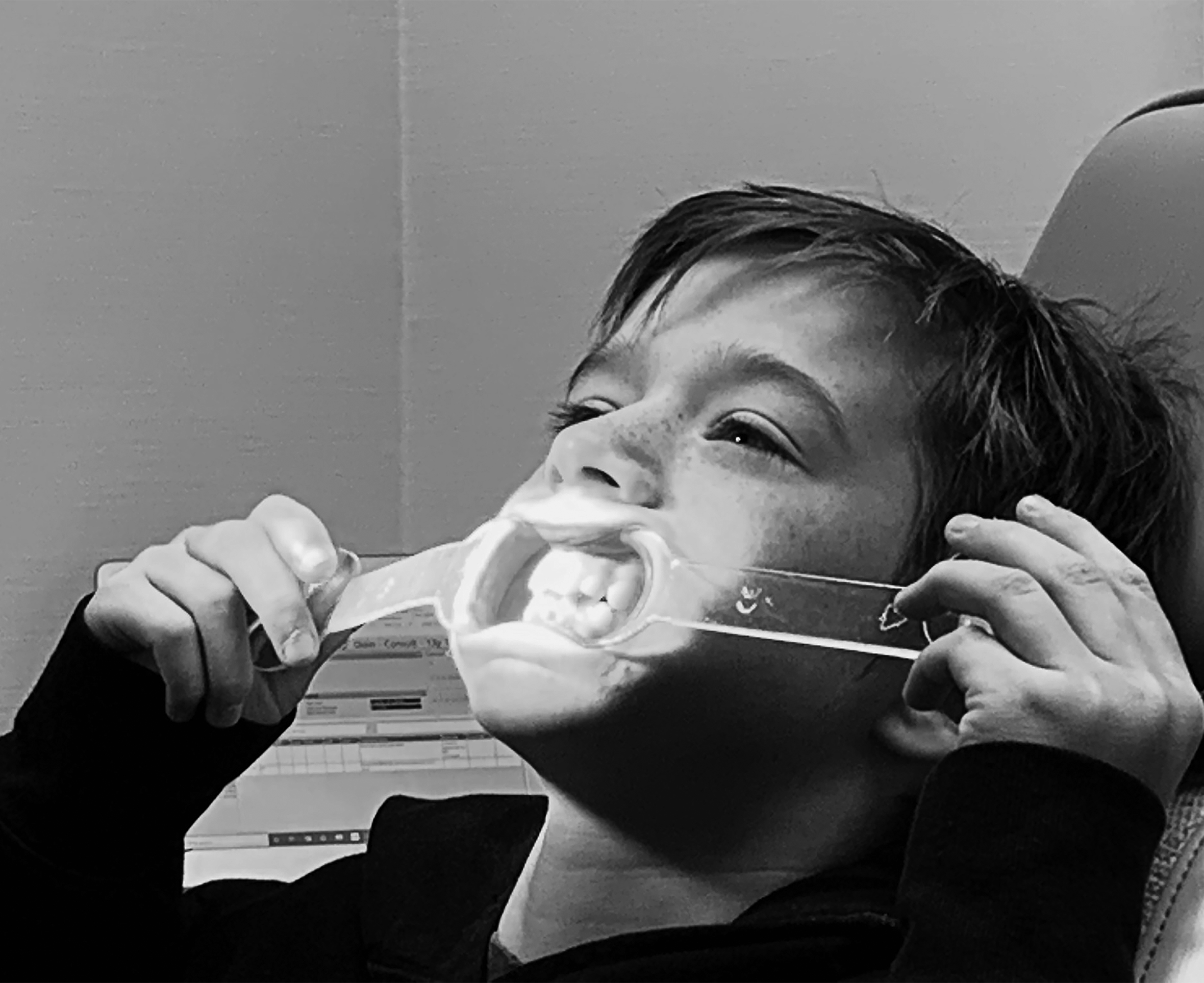The black and white photograph captures a young boy, around 11 or 12 years old, seated in a dentist's chair, identified by the overhead illumination commonly used in dental examinations. The boy has short brown, scraggly hair and freckles dotting the bridge of his nose and cheeks. He wears a long-sleeved shirt or hoodie and seems calm, though slightly uncomfortable, as he tilts his head back. He holds two handles attached to a piece of plastic, likely a mouth spreader, that stretches his lips, revealing his teeth. His glimmering eyes and the precise detailing of his face make the scene vividly striking.